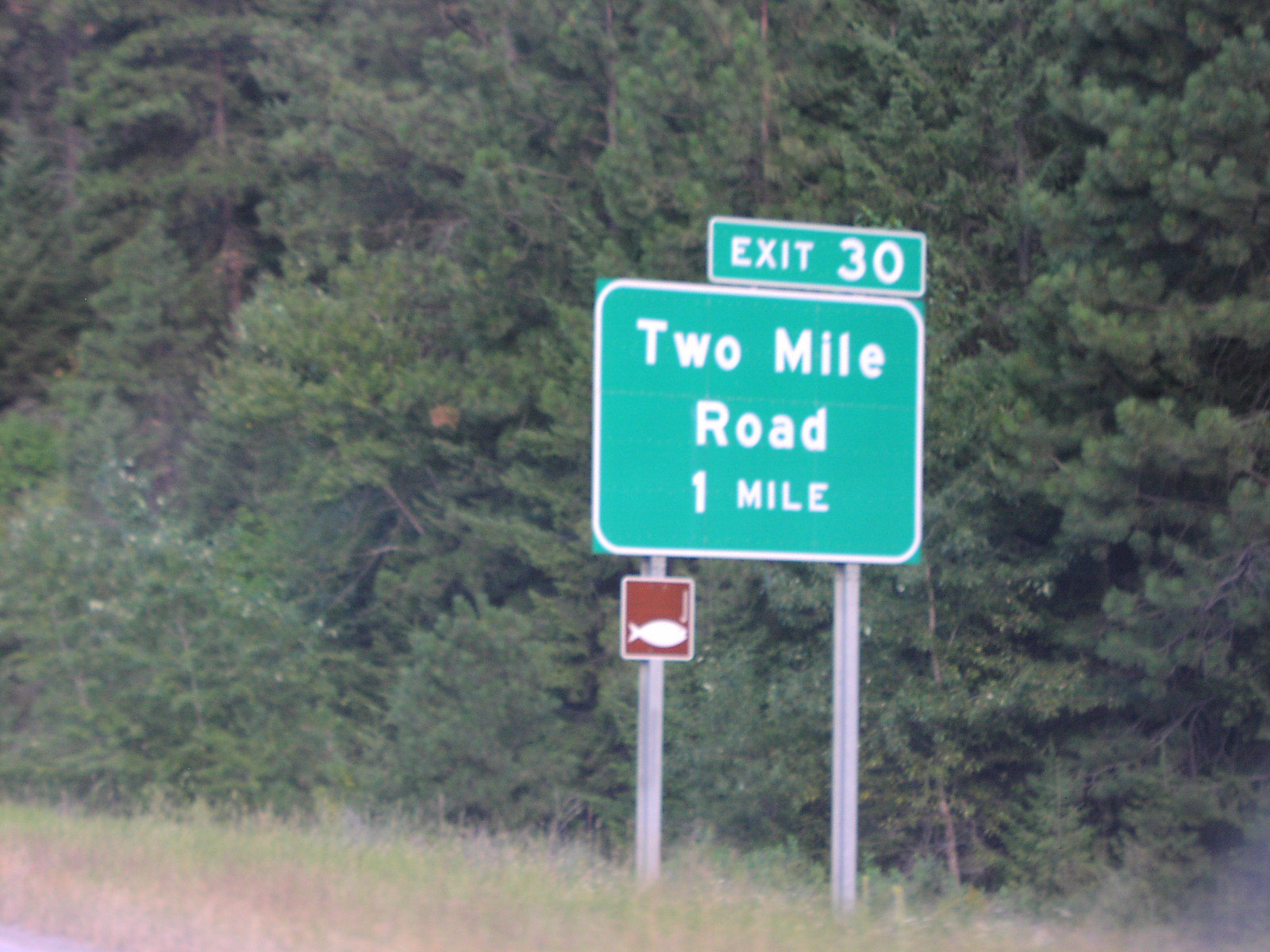In the image, the foreground features a patch of dry grass. Rising from this are blue-silver metallic arms and legs, with a noticeable metal leg on both the left and right sides. On the left side of the scene, there's a red sign displaying a white fish emblem. Above this is a larger green sign that includes a rectangular white board with the text "2 mile road to 1 mile." In the top right corner, a smaller square sign reads, "I got a bit dirty." The background shows a lush expanse of green trees, their branches extending outward and adorned with fine leaves. The bottom left corner of the image includes a mix of green and brown tones, with visible branches and bark providing additional texture.